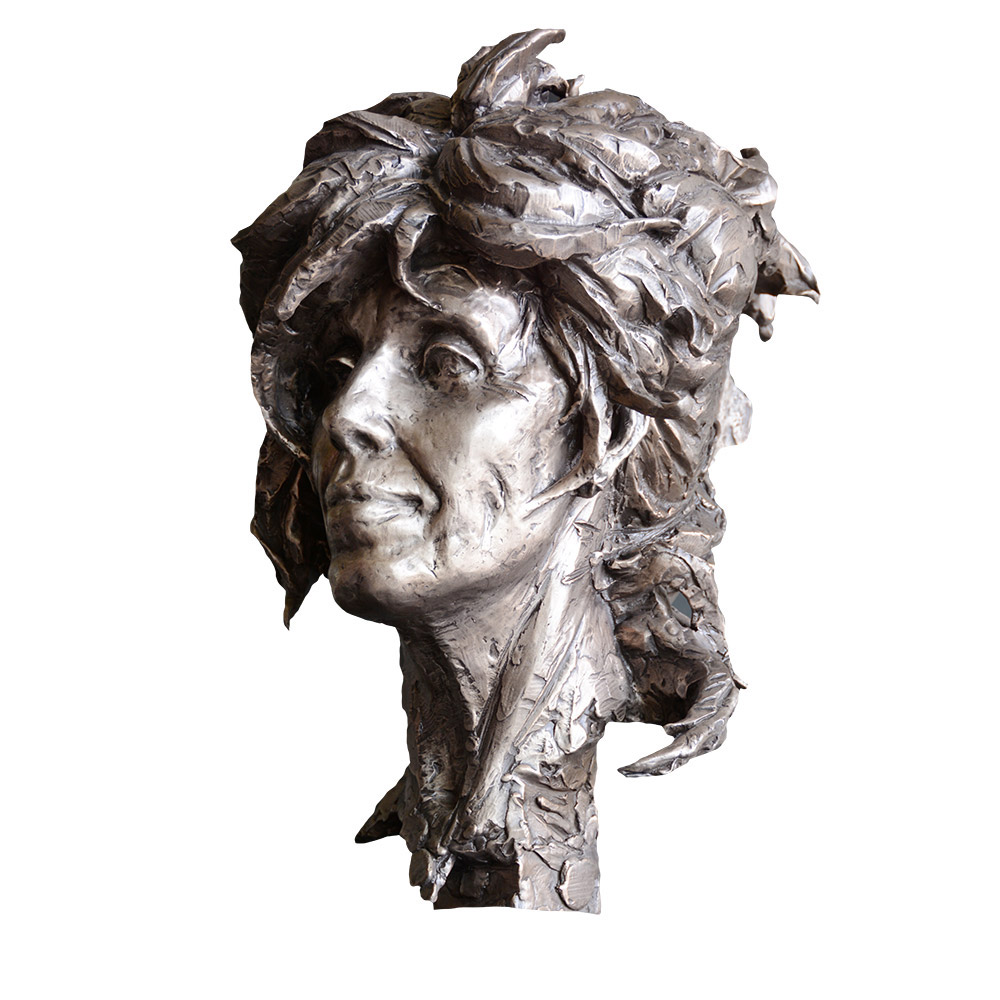This photograph showcases a detailed bronze bust of a woman, set against a completely white background. The sculpture, made of a shiny brownish metal likely bronze, features intricate details and a stylized aesthetic. The neck appears quite angular and sharp, with visible chips where the material has been worked, giving a textural quality to the bust. The woman portrays a smiling expression, with slightly indented cheeks and hooded eyes. Her earlobes are exaggeratedly attached to her face via long flanges. 

The full, thick hair of the sculpture is notably intricate, with exaggerated clumps and sections pointing in various directions. Some strands are curled, including a small fringe that curls down over her left eye, while others are straight, surrounding her face and extending halfway down her neck. Despite the precise and elaborate detailing, the sculpture appears to be missing part of the neck, suggesting it might have originally been part of a more extensive piece. The woman’s strong jawline, regular-sized nose, full lips, and slightly inset eyes contribute to the suggestion she may be an important historical figure, though her exact identity, race, or ethnicity remains unspecified. The overall impression is of a dignified and possibly mature woman with an expressive, stylized portrayal.